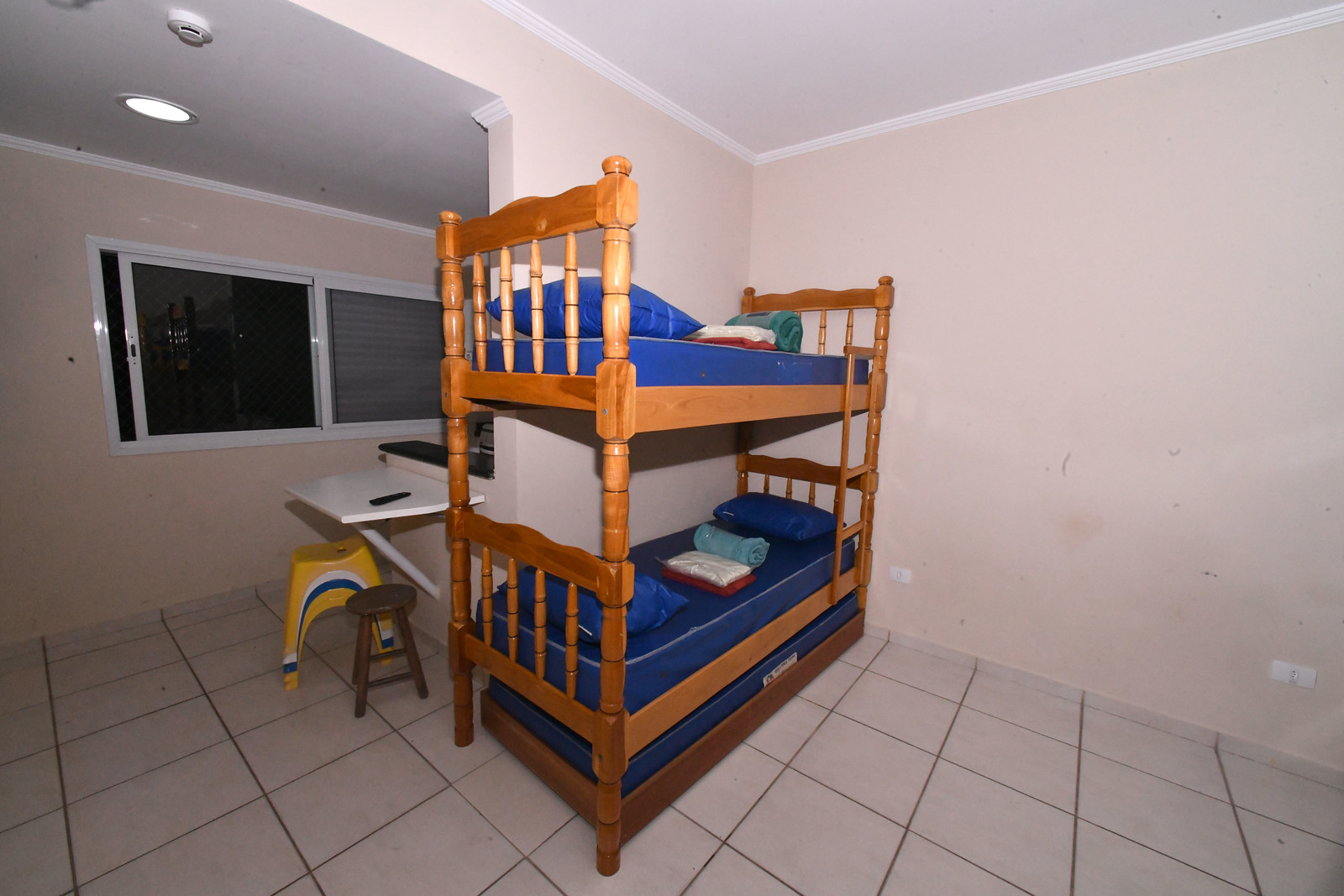The image depicts a bedroom with beige walls and a white ceiling. The flooring consists of large square white tiles. In the top-left corner of the room, a recessed light fixture is mounted on the ceiling. Against the left wall, there is a slightly open sliding window, revealing a night scene outside; one pane is pushed to the right, and the right window has a blind.

In the corner of the room stands a wooden bunk bed with spindle-style frames. Each bunk has blue bedding, blue pillows, and folded sheets in white, red, and green. A wooden ladder is attached to the frame, providing access to the upper bunk. Beneath the lower bunk, there appears to be a trundle bed with matching blue bedding.

Next to the bunk bed, a simple white desk is mounted to the wall, supported by a singular pole. Under the desk, there are several plastic stools stacked in yellow, white, and blue colors, along with a separate brown stool nearby. The walls show slight signs of dirt, and there are several white electrical outlets visible.